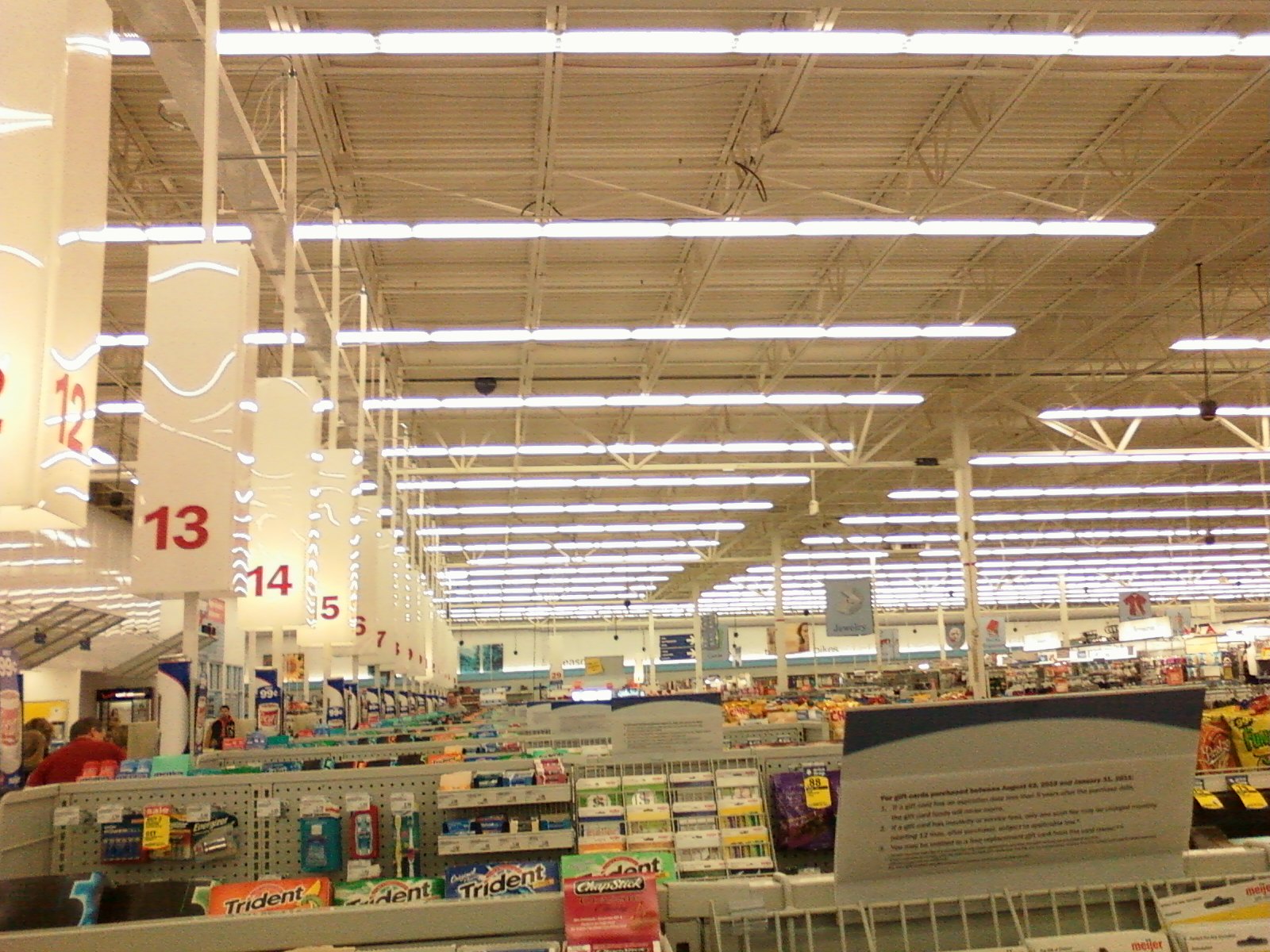The image is a detailed color snapshot taken inside a large supermarket, showing the checkout aisles stretching from number 12 onward, clearly visible and labeled with large, rectangular illuminated signs mounted on white posts. 

The snapshot captures aisles up to number 25, indicating a ton of checkout lanes, yet only about five of them have their lights on, suggesting they are the only open ones. The store's ceiling reveals exposed beams and wiring, indicating a metal frame structure, and it's brightly lit with long, tube-like fluorescent lighting. 

The foreground prominently features a shelf with grab-and-go items typical of a checkout area, including several packs of Trident chewing gum in blue, green, and orange varieties, all marked with large text. Additional items on the shelves include possible grab-and-go medicine like allergy meds, aspirin, hand wipes, Funyuns, and Cheetos, further emphasizing the impulse shopping setup. While the main store area in the background shows more department signs, they are too distant to read clearly.